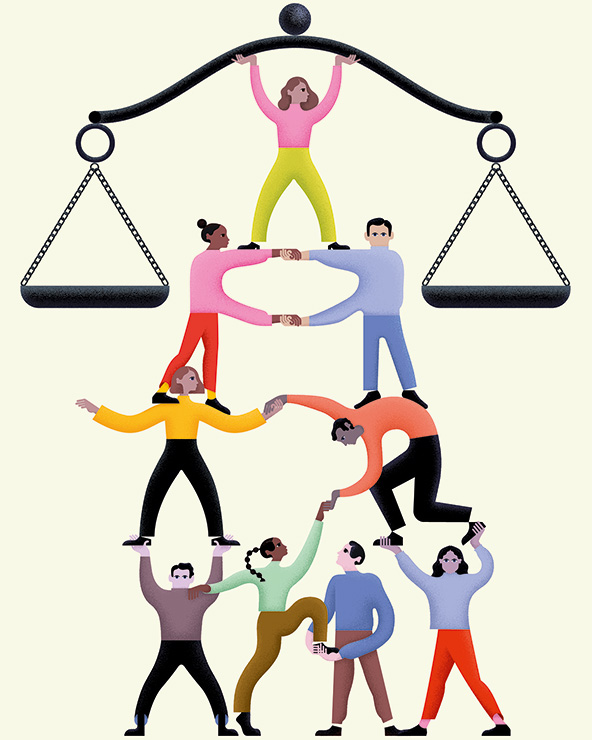The image is a detailed drawing of people forming a human pyramid on a white background. At the bottom layer, there are four individuals, each contributing to the stability of the structure. Among them, a woman in orange pants and a lavender sweatshirt is holding up a man dressed in black pants and an orange shirt. Another man, wearing blue pants and a light blue sweatshirt, stands on the previous man's back, holding hands with a woman in a pink sweatshirt and orange pants. The pyramid continues to rise, culminating with a woman at the top, standing on the interlocked arms of the two beneath her. She is dressed in light green pants and a pink sweater, and is holding up a scale reminiscent of the Our Lady Justice statue. The scale features a base with open triangles on each side, a curved bar, and a decorative black ball on top. The drawing represents nine stylized characters in total, forming an intricate and balanced human structure.